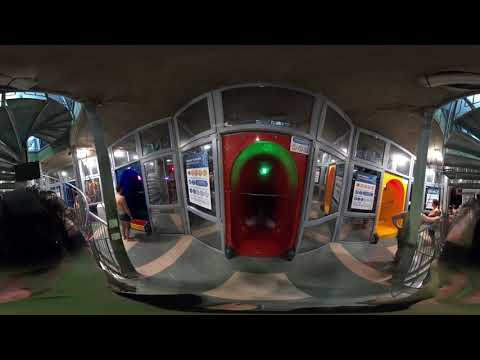The image depicts a vibrant entertainment area, possibly a children's play zone, surrounded by metal-framed, see-through glass walls. Centrally positioned is a distinctive red door with a blackish handle set in the middle, topped by a circular green light. This red door is accented by red and green hues around its frame, and a small white sticker with blue text is placed in the top right corner of the door. To the immediate left of the door, there is a large poster with three rows of colorful boxes: blue and white on the bottom, all blue in the middle, and orange on the top. Further to the right within the room, another similar poster can be seen beside what appears to be an orange and yellow entrance.

Two individuals are observed outside, examining the area, and a shirtless man gazes into a blue entrance on the far left, which features a red and yellow staircase below it. Additionally, a spiral staircase is present on the far left, ascending to the building's top. The scene is awash with a plethora of colors including teal, green, white, blue, red, and yellow, enhancing the playful atmosphere. Although the exact function of the different tunnels and entrances remains unclear due to their darkened interiors, they hint at a possible adventure and exploration theme. The overall setting suggests a lively and engaging space designed for fun activities and adventures.